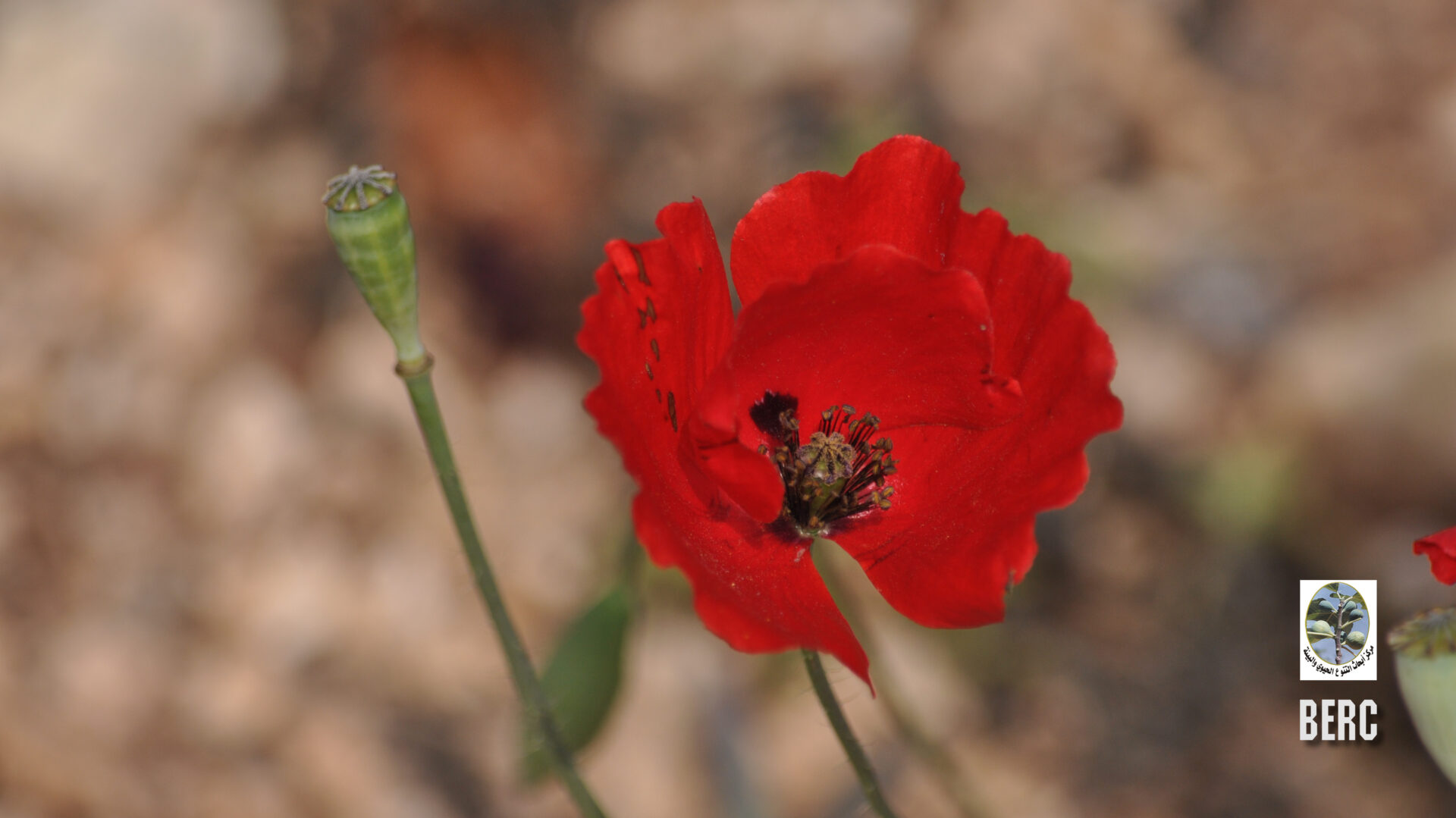This detailed color photograph prominently features a zoomed-in red wildflower with large, partially separated petals. The photograph is taken from an angle that looks down into the flower, highlighting its intricate details. The flower's center reveals stamen with dark brown filaments. The vibrant red petals contrast sharply with the thin green stalk supporting the flower. To the left of the main flower, another green stalk supports an upside-down, dome-shaped green bud, indicating a flower that has not yet bloomed. The background is notably blurry and blotchy in shades of brown, emphasizing the close-up nature of the shot and the limited depth of focus. In the bottom right corner, the image features a logo with a white background and an oval picture, accompanied by black text in a foreign language. Below the logo, in large white letters, are the initials "B.E.R.C."